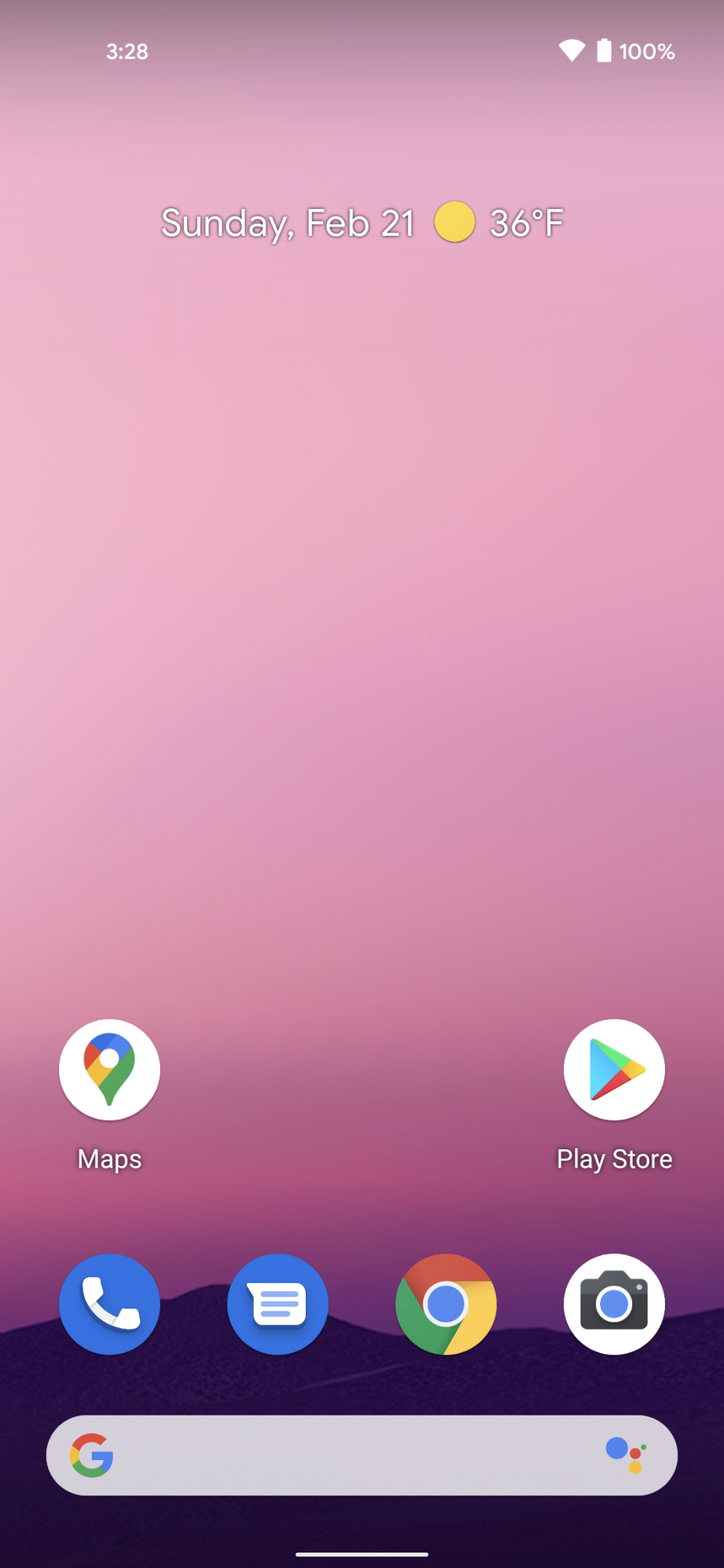The image depicts a phone's vertical screen with a pink background. In the top-left corner, the time is displayed as 3:28 in white text. Moving to the top-right corner, the Wi-Fi icon indicates a connected internet status, and the battery indicator shows 100% charge. At the center-top, the date is denoted as "Sunday, February 21." Below the date, a yellow circle icon signifies the weather, displaying "36°F." 

Towards the bottom of the screen, the first row features app icons: "Maps" on the far left, and "Play Store" on the far right, with considerable space between them. Directly below the "Maps" icon is an image of a blue circle with a white phone symbol. In the same row, sequentially from left to right, are the icons for messaging (a blue circle with a text bubble), the Chrome browser, and a white circle with a camera icon.